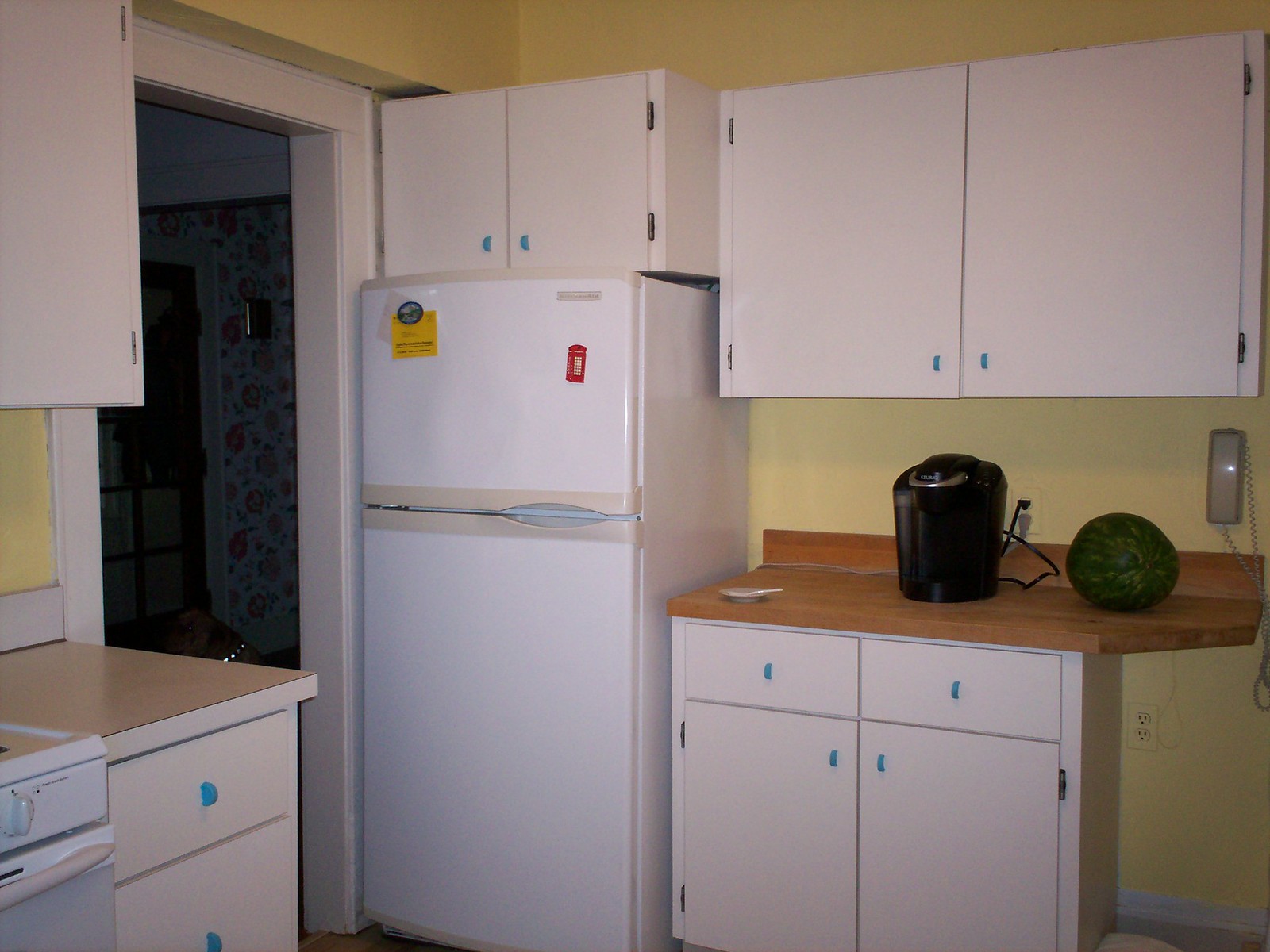This photograph captures a nostalgic, outdated kitchen, enclosed and compartmentalized, suggestive of a 90s apartment. The walls are painted a warm yellow hue, contributing to the vintage ambiance. Central to the image is a small, white, top-and-bottom loading refrigerator adorned with a red English phone booth magnet and a blue circular magnet holding a yellow paper. Flanked around it are two ground-level cabinets with reddish-brown wood laminate countertops and two matching overhead cabinets.

To the left of the fridge, a doorway with a white frame leads to another room, displaying floral wallpaper with red, green, and yellow flowers, and part of what appears to be a brown shaggy dog with a studded collar. Adjacent to the fridge on the right, the countertop hosts a black single-cup Keurig coffee maker with a silver handle and a whole watermelon, with a beige corded phone mounted above on the wall.

Further to the right, there's more counter space with a white laminate countertop, revealing two drawers donning unique, semi-circle, aqua blue plastic handles. The lower cabinet hardware matches this distinctive style. Just visible is the edge of a white stove, showcasing its white dial and handle. The overall aesthetic of the kitchen resonates with a budget-conscious design, reinforced by the modest materials and retro fixtures.